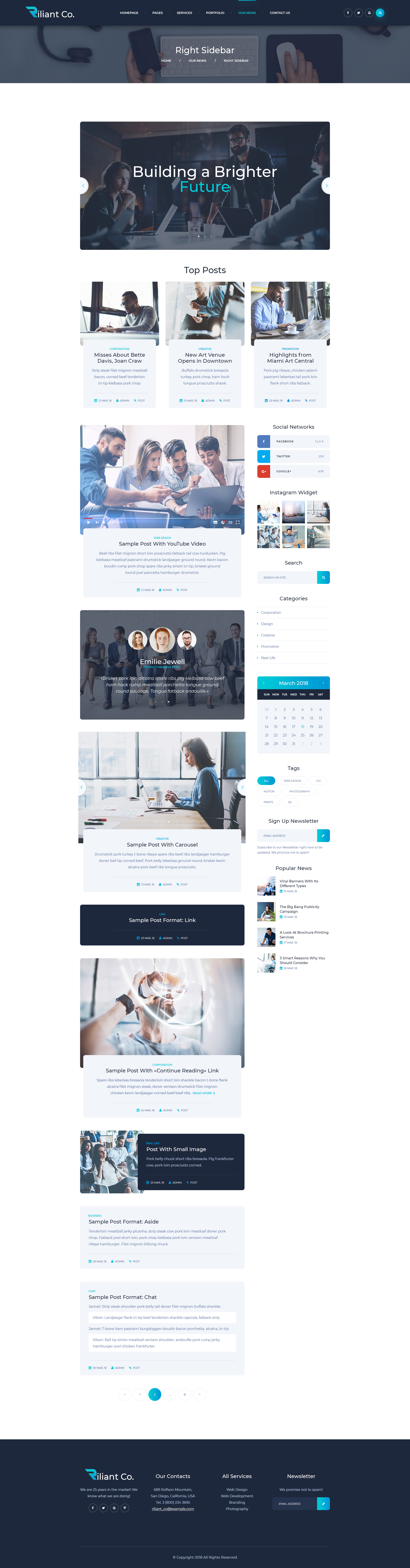This screenshot presents a distorted, low-resolution image of a website, likely a landing page, compromised by a squished aspect ratio that causes circular elements to appear oval and text to be difficult to read. 

The top menu bar is shaded in a dusky dark blue, giving a sophisticated tone to the website. Below, a translucent blue overlay partially masks the main visual, which features an individual seated at a keyboard. This person is holding a phone in the left hand and manipulating a white mouse with the right hand. Despite the poor resolution, white text is visible but mostly illegible.

Prominently, a banner at the top of the page reads "Building a brighter future," with "building a brighter" in white and "future" in teal, set against an image of people gathered around a meeting table. Additional stock images and linked sections, presumably featuring professional photographs, showcase people around a laptop and individuals at workstations, possibly leading to their profiles or related content.

The sidebar suggests options for sharing and includes a calendar function alongside links to other articles. The website's footer mirrors the dusky dark blue theme, again featuring white text that remains challenging to decipher due to the poor resolution and distortion.